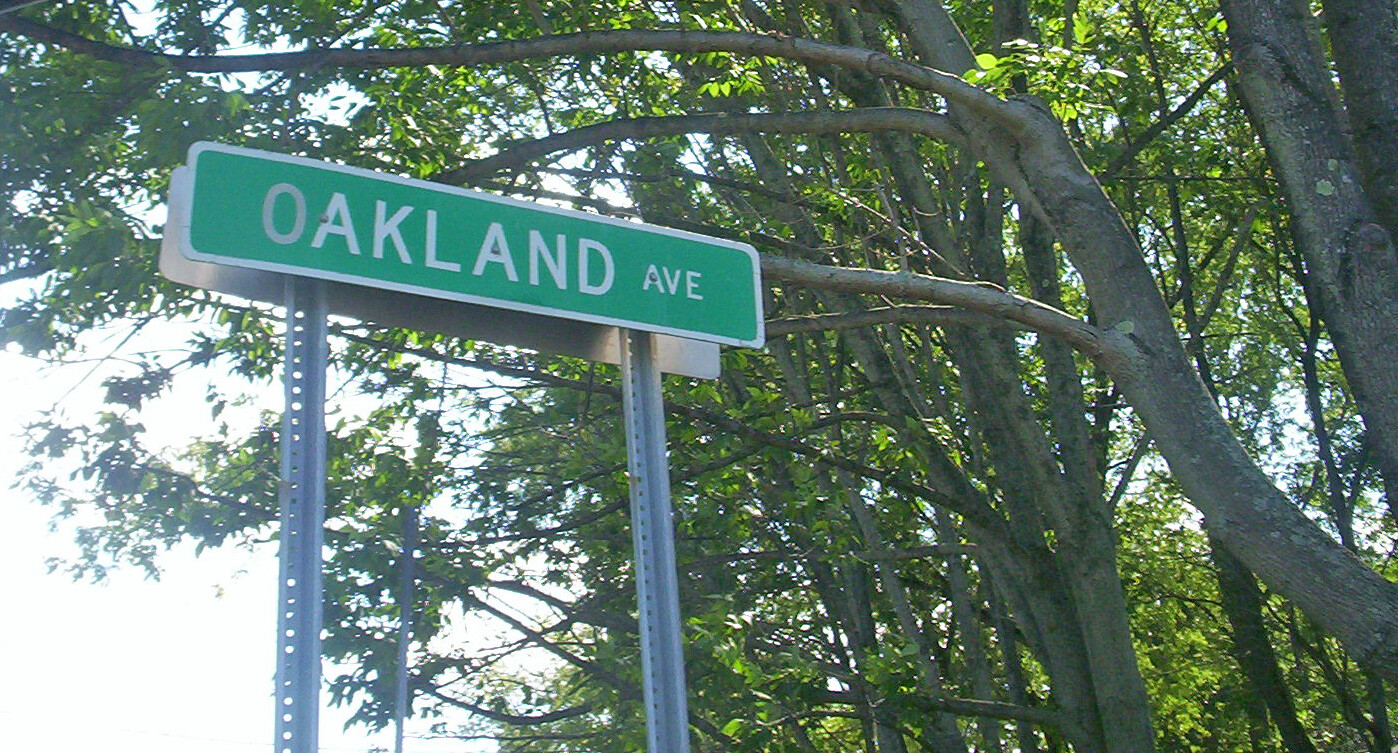This daytime outdoor image captures a bright and sunny scene featuring a street sign for Oakland Avenue. The sign, rectangular in shape with a green background, displays "Oakland Ave" in white letters and is securely mounted on two drilled, metal posts. Positioned on the left side of the horizontal image, the sign is viewed from below, angled upwards towards the sky, which appears pale blue, suggesting a potentially cloudy day. The backdrop consists of several healthy, leafy deciduous trees with abundant green foliage and sturdy trunks. The trees' branches are spread across the right to left side of the image, appearing to bend as if swayed by the wind. No other man-made objects are present, creating a harmonious blend of natural elements and street signage.